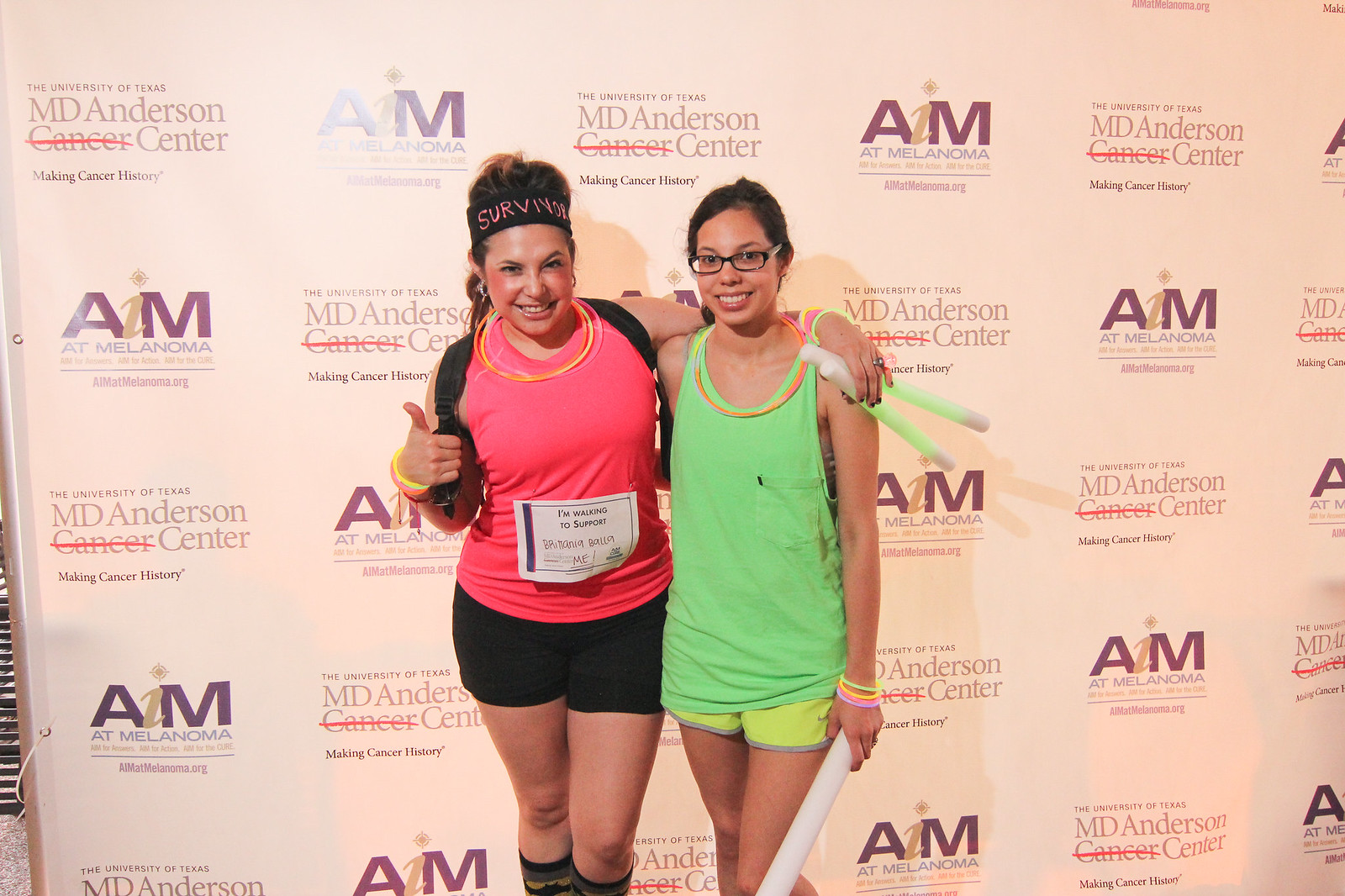In front of a backdrop featuring the logos for AIM at Melanoma and MD Anderson Cancer Center, with the slogan "Making Cancer History" and the word "cancer" crossed out, two women pose proudly after completing an athletic event. The woman on the left, wearing black shorts and a hot pink tank top reminiscent of bubble gum, sports a headband that reads "Survivor" in pink letters, with her hair tied back in a ponytail. She has a thumbs-up gesture, a substantial amount of blush on her cheeks, glow bands, necklaces, and an identification tag on her stomach. She appears to be slightly older and may have a backpack on her back. Her companion, to the right, is dressed in a lime green tank top with yellow shorts. She has brown hair, black glasses, and a bright smile, accessorized with glow bands on her wrist and neck. She holds a rolled-up poster or a white baton in her left hand. Both exude a sense of accomplishment and camaraderie, embodying the spirit of the event they have just completed.